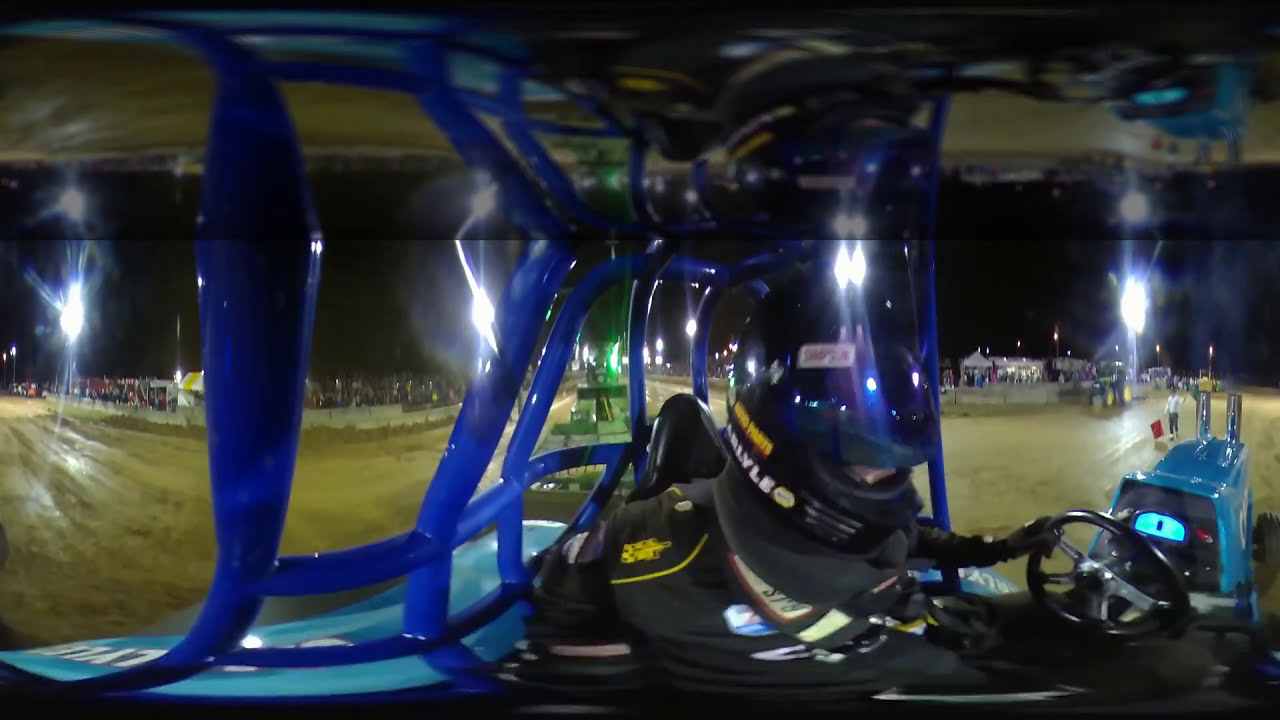The photograph captures a dramatic night-time scene of a race car driver navigating a muddy racetrack. The image is taken in a panoramic style, resulting in a slightly distorted, elongated view. The central figure is clad in a full black motocross outfit and a shiny black helmet, seated in the cockpit of a race car surrounded by a neon blue cage-like structure. The driver grips a black steering wheel located in the bottom right corner of the image. Behind him, the racetrack is depicted as a dirt-covered, W-shaped terrain, leading up to a backdrop of darkness punctuated by the glow of five large white lights and numerous smaller ones. Adding to the atmospheric tension, a few tiny figures of spectators can be seen in the distance, positioned under the vast, night sky. The blue gauges inside the vehicle are faintly illuminated, emphasizing the high-tech setting of this intense racing moment.